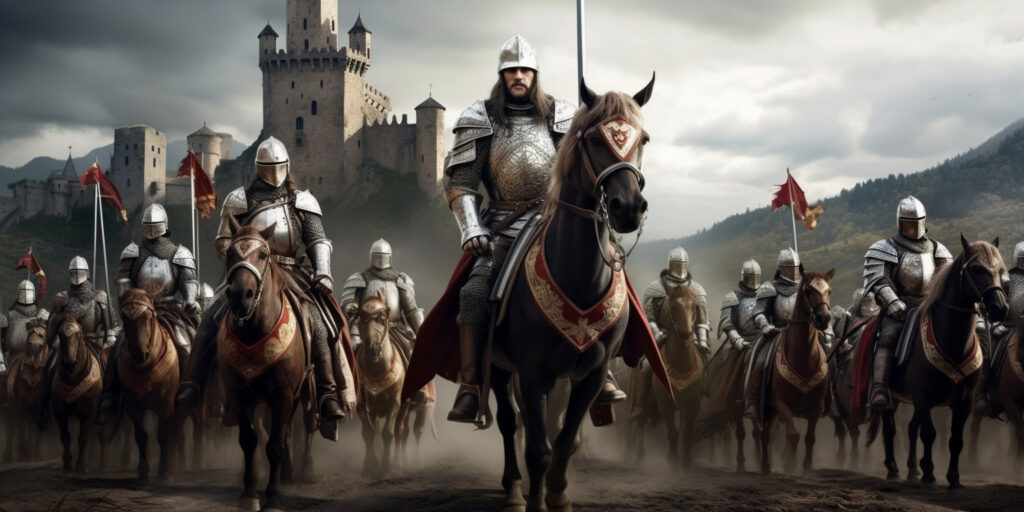The painting depicts a group of around fifteen medieval knights clad in shiny, stainless steel armor, riding brown horses. The knights, all facing forward as if preparing to advance, are arranged in a spread-out formation, seemingly getting ready to march or head into battle. The central figure, who appears to be the leading officer, is distinguishable by his visible face, featuring a curly mustache and long brown hair. The knights are holding up red and yellow flags, with one particularly prominent individual raising a sword. The backdrop features a tall, luxurious stone castle with spires, set against gray, overcast skies. In the distance, there are mountains adorned with trees. The overall palette of the painting includes a lot of beige and gray tones, with striking highlights of silver from the armor and red from the flags. Dirt trails in the air enhance the dynamic movement of the scene, adding to the sense of imminent action.